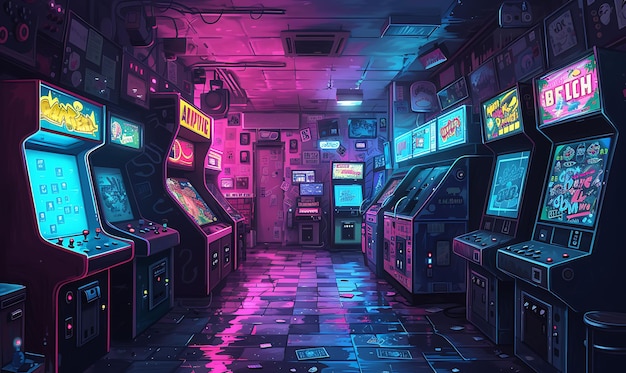The image depicts a detailed, immersive scene of a futuristic or sci-fi inspired arcade, possibly an artistic render rather than a photograph. The setting is bathed in ambient lighting with a distinctive pinkish-purple light reflecting off the shiny black tiled floor. On the left side, there are four arcade machines displaying vibrant, multicolored hues of yellow, blue, green, and purple; these include two standard-sized cabinets, one double-wide machine, and another standard one. The right side features another set of four arcade machines – two standard and two double-width – adjacent to an additional machine with a blue screen. The arcade's atmosphere is dark and seemingly devoid of people, similar to a scene after closing hours, highlighting the glowing neon hues of pink on the left and blue on the right, creating a striking visual divide down the center. The text on the screens appears illegible, resembling AI-generated fonts, adding to the futuristic feel. The exaggerated and colorful titles of the games hint at classic arcade aesthetics, despite the overall setting suggesting a more contemporary or speculative design.